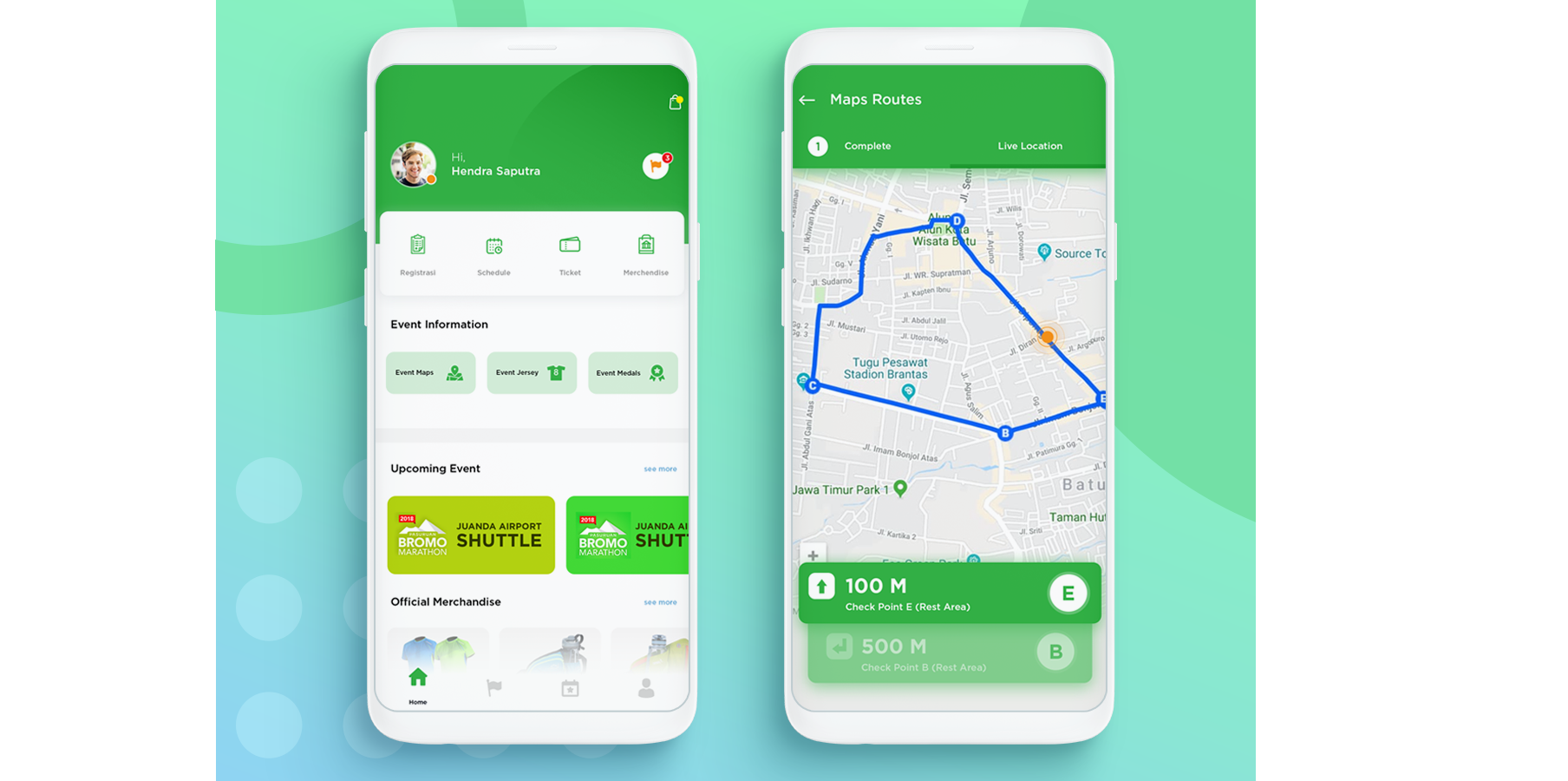The image features a turquoise teal-colored background with two smartphones displayed side-by-side. 

**Left Smartphone:**
- The top section features a green header reading "Hi Hendra Saputra".
- Below the header, there are four distinct buttons/options. The first button says "Ticket", while the second button is not clearly described. 
- Below these buttons, there is a section titled "Event Information" which contains three gray boxes, each with a symbol and text inside.
- Further down, an area labeled "Upcoming Event" displays two boxes:
  - The left box is yellowish-green and labeled "Bromo Marathon Juanda Airport Shuttle".
  - The right box is lime green, containing the same text.
- At the very bottom, there is a section labeled "Official Merchandise".

**Right Smartphone:**
- Shows a header that reads "Map Routes".
- Below the header, there is an image of a map with a highlighted green route indicating a specific path or direction.